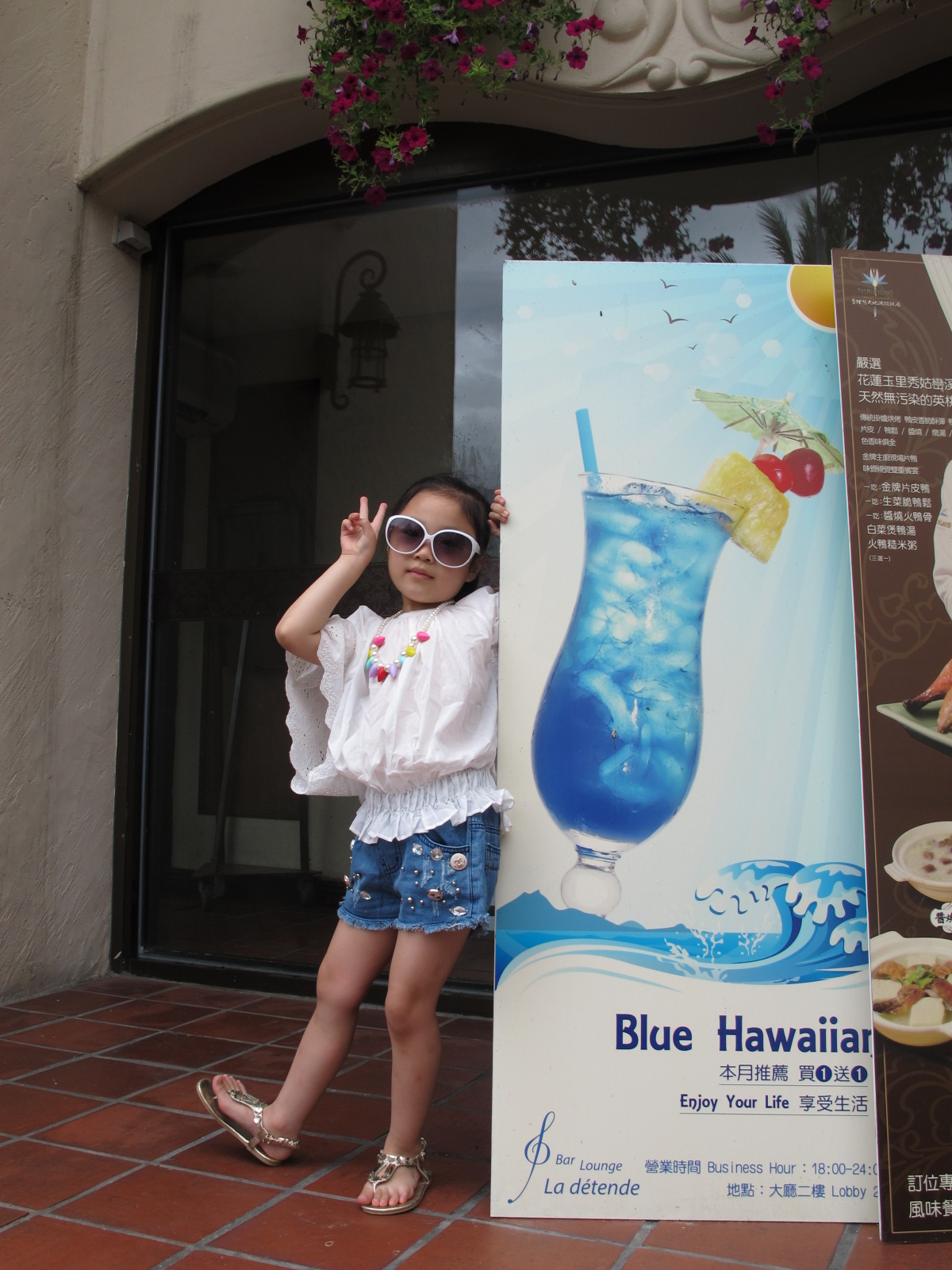In this vibrant outdoor photo, a little girl with light skin and very dark, almost black hair stands as the central focus, exuding a playful charm. She is dressed in white sunglasses, a baggy white blouse adorned with a colorful neckline featuring pink, red, yellow, blue, and white accents, blue jean shorts, and golden sandals. Striking a fun pose, she raises her right arm to show a peace sign beside her head while her left hand is on a poster sign. The poster, nearly a foot and a half taller than her, features a refreshing image of a blue tropical drink with a blue straw, a pineapple with cherries on the side, an umbrella, and a wave design underneath. The text "blue Hawaiian" is prominently displayed at the bottom, with additional Chinese characters that read "enjoy your life." She stands in front of a glass entrance with red-orange tiled flooring, likely belonging to a restaurant, adding to the lively atmosphere of the setting.